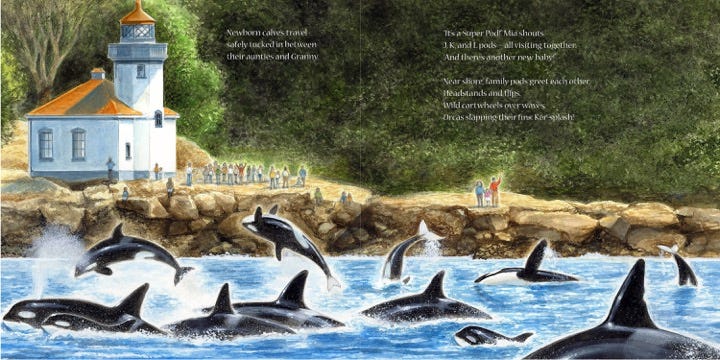In this vivid outdoor scene, a white cement building with an orange roof and attached tower, possibly a lighthouse, stands prominently. The tower features a balcony encircled by a gray fence. The structure is set against a lush backdrop of green trees with varying shades of light and dark green. In front of the building, a large body of water teems with activity. Numerous orcas, identifiable by their distinct black and white coloration, are seen leaping and swimming, creating dramatic splashes as they move in and out of the blue water. The shore is a mosaic of tan, brown, and black rocks where a crowd of people has gathered. Among them, a family with a man, a woman, and a girl in blue, pink, and orange can be seen waving enthusiastically. The image also includes some white text detailing the behavior of the orcas: "newborn calves travel safely tucked in between their aunties and granny," and mentions of family groups greeting and performing flips over waves. The overall atmosphere is dynamic and vibrant, capturing the natural beauty and interaction between humans and wildlife.